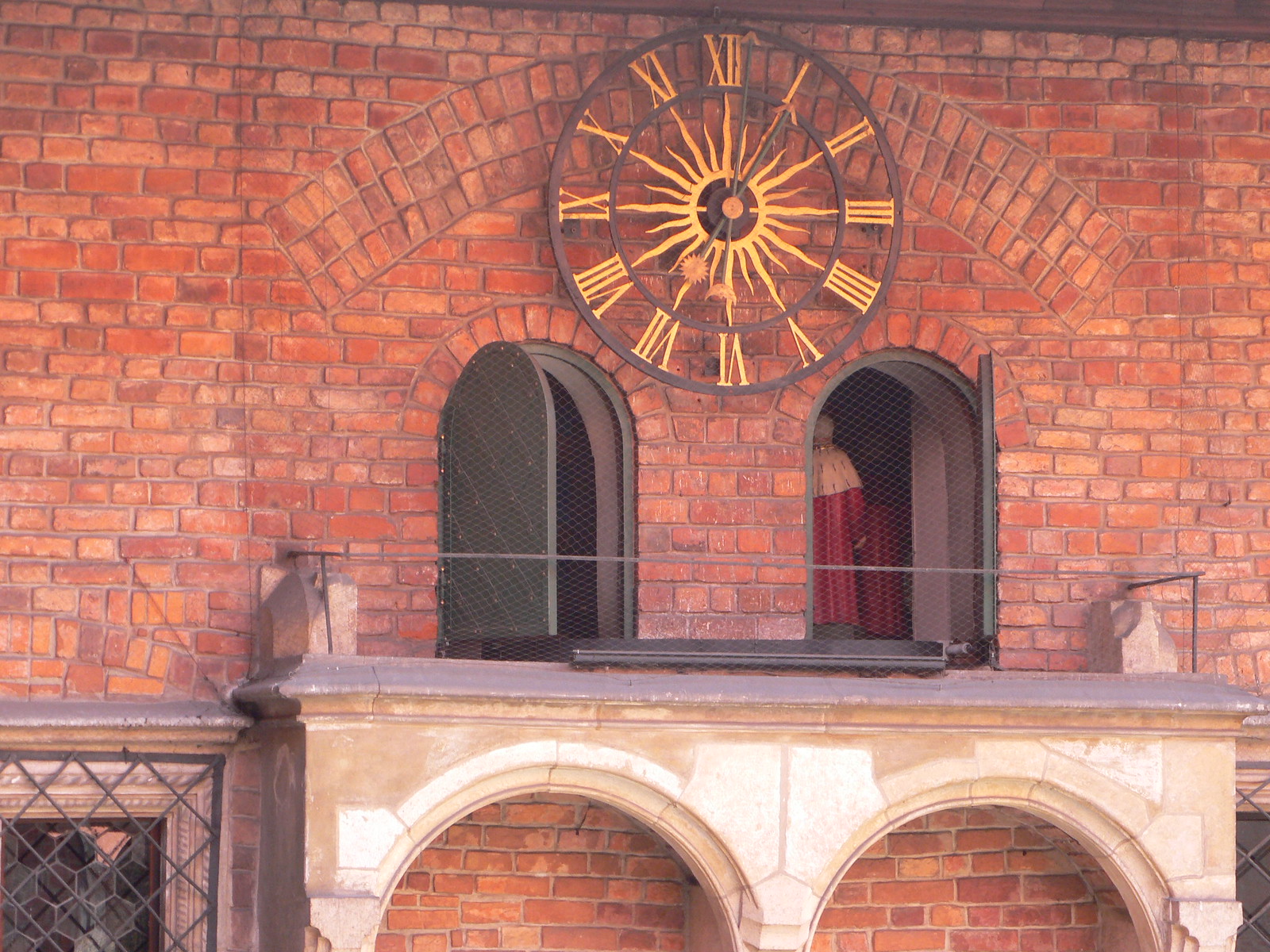The outdoor photograph captures a detailed and historic scene centered around a prominent clock on the upper section of a red brick wall. The background, composed of various shades of reddish-brown bricks with some lighter orange and white markings, holds a round clock with a black wrought iron frame. This clock features gold Roman numerals and a striking gold sunburst design at its center. The hands of the clock, which point to one o'clock, are intricately designed, resembling a sun and a crescent moon.

Directly below the clock, integrated into the brickwork, are two arched openings with metal doors - one swinging left and the other right. These doors, made of black or brown metal, reveal small figures resembling a man with gray hair, dressed in a red robe with white trim. These figures suggest a German-style clock mechanism that displays figurines at specific times.

Supporting the structure beneath the openings is a light gray-tan stone porch, upheld by two elegant arches. Through these arches, more of the red brick wall can be seen, along with a window on the left that is covered by black grating. The detailed craftsmanship of the clock and the architectural elements add to the photograph's historical and artistic charm.